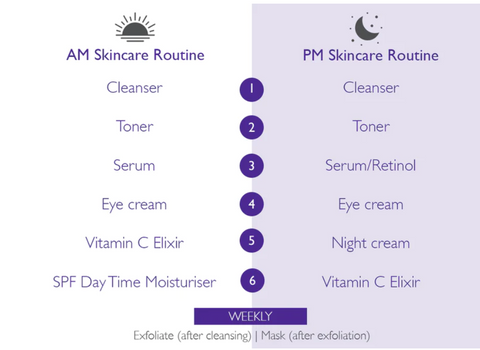The image is a detailed graphical chart outlining a skincare routine, split into two halves for AM and PM routines. On the left side, labeled "AM Skincare Routine" with an icon of a rising sun over water, there's a vertical list against a white backdrop featuring the steps: cleanser, toner, serum, eye cream, vitamin C elixir, SPF, and daytime moisturizer. On the right side, under "PM Skincare Routine" accompanied by a moon and stars icon, the routine is listed on a purple backdrop and includes: cleanser, toner, serum, retinol, eye cream, night cream, and vitamin C elixir. Down the center, connecting both halves, are numbers 1 to 6 indicating the order of steps. At the bottom, a purple banner with white writing provides weekly instructions: "Exfoliate after cleansing and mask after exfoliation." The overall design uses clean, sans-serif fonts, with mostly purple lettering and darker purple numbers to delineate steps.